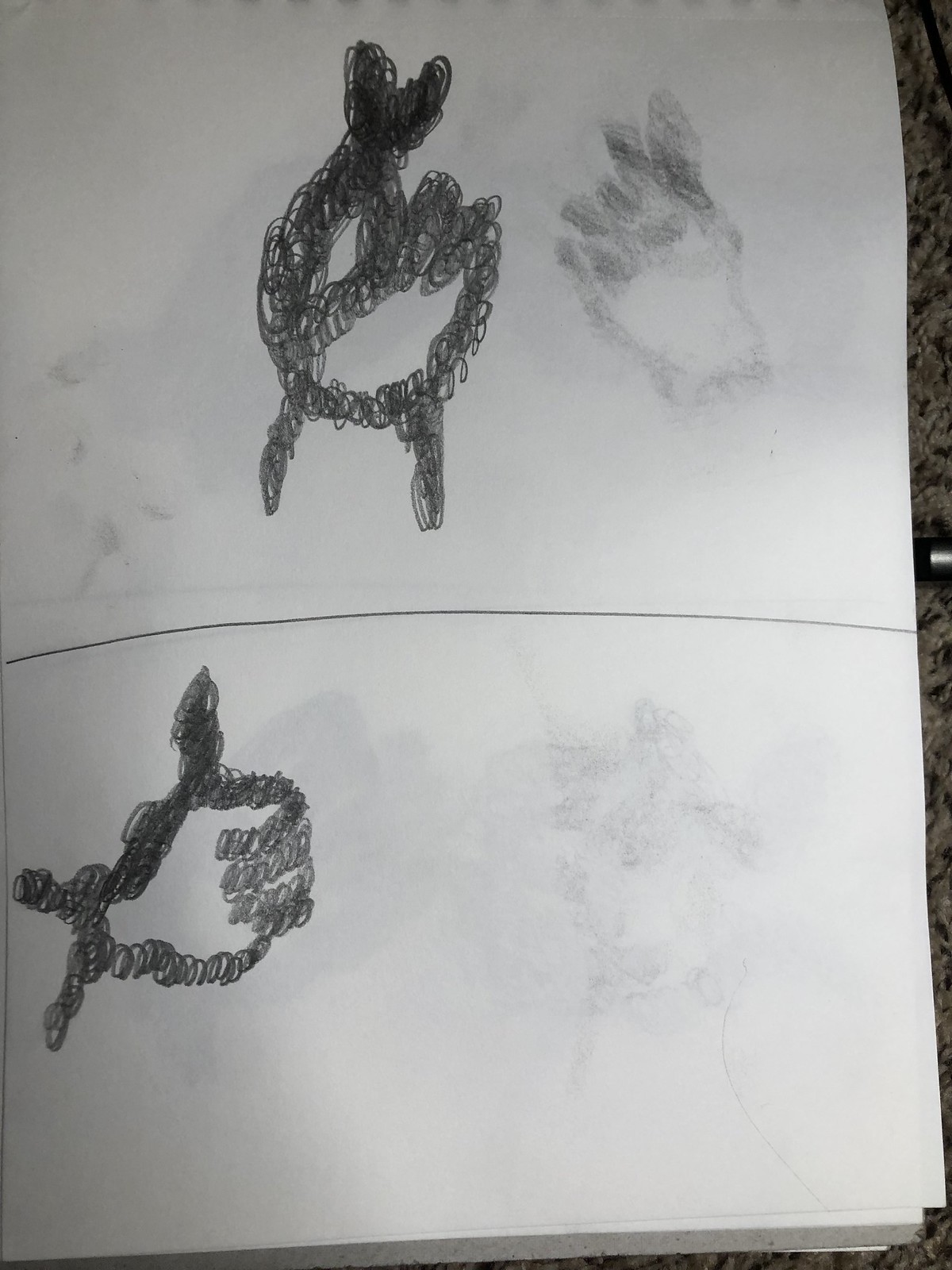In this image, we see a piece of white paper, likely from a notebook or sketchbook, with its top edge slightly crinkled upward. The paper is divided into two sections by a line drawn just below the midpoint. On the top section, there is a pencil or pen drawing that appears to depict a hand with the index and middle fingers crossed. The drawing is composed of very dense, circular squiggles, making the image somewhat abstract and giving it a vague, sketchy appearance. The thumb of this hand is drawn along the side, but the overall outline remains ambiguous due to the dark, almost black loops of pencil.

In the bottom section, another hand is drawn in the same dense, circular squiggle style. This time, the hand is more clearly defined, with the thumb pointing upwards in a 'thumbs up' gesture. The fingers are more recognizable in this drawing, although the thumb is depicted as a solid black blob, reinforcing the abstract style.

The paper rests on a marble countertop that is partially visible on the right edge of the frame. A pen is positioned horizontally along the counter. The entire notebook occupies most of the frame, lending a simple yet detailed context to the scene.